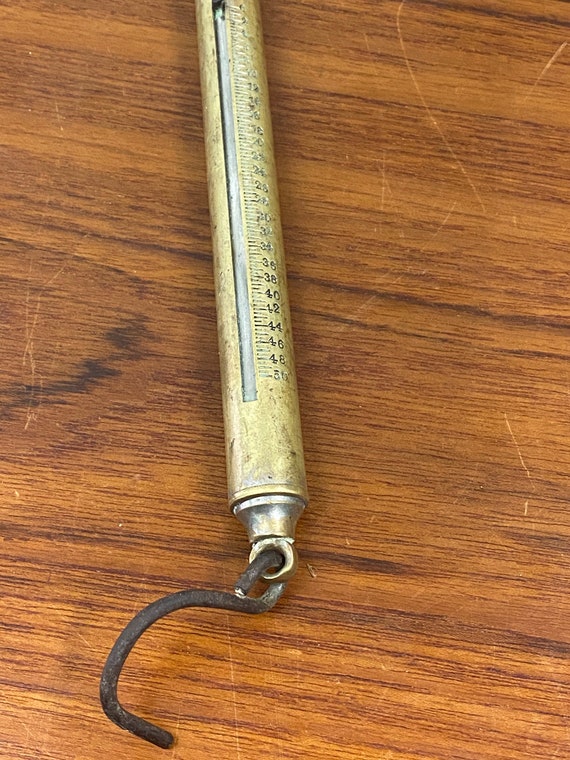The image features an antique, narrow, cylindrical brass scale resting on a scratched wooden surface, possibly a table. The metallic tool, reminiscent of bronze, is characterized by a vertical cutout running along its length, revealing a white band inside. The scale has measurement markings running from five to one, suggestive of gauging weight or pressure. It also includes an old, rusty metal hook at the bottom, which might have been used to hang the tool for storage. The hook connects through a loop at the end of the stick, adding to the vintage aesthetic of the instrument. The intricate details, such as the worn-out appearance and the visible wood grain background, enhance the historical and functional context of this measuring device.